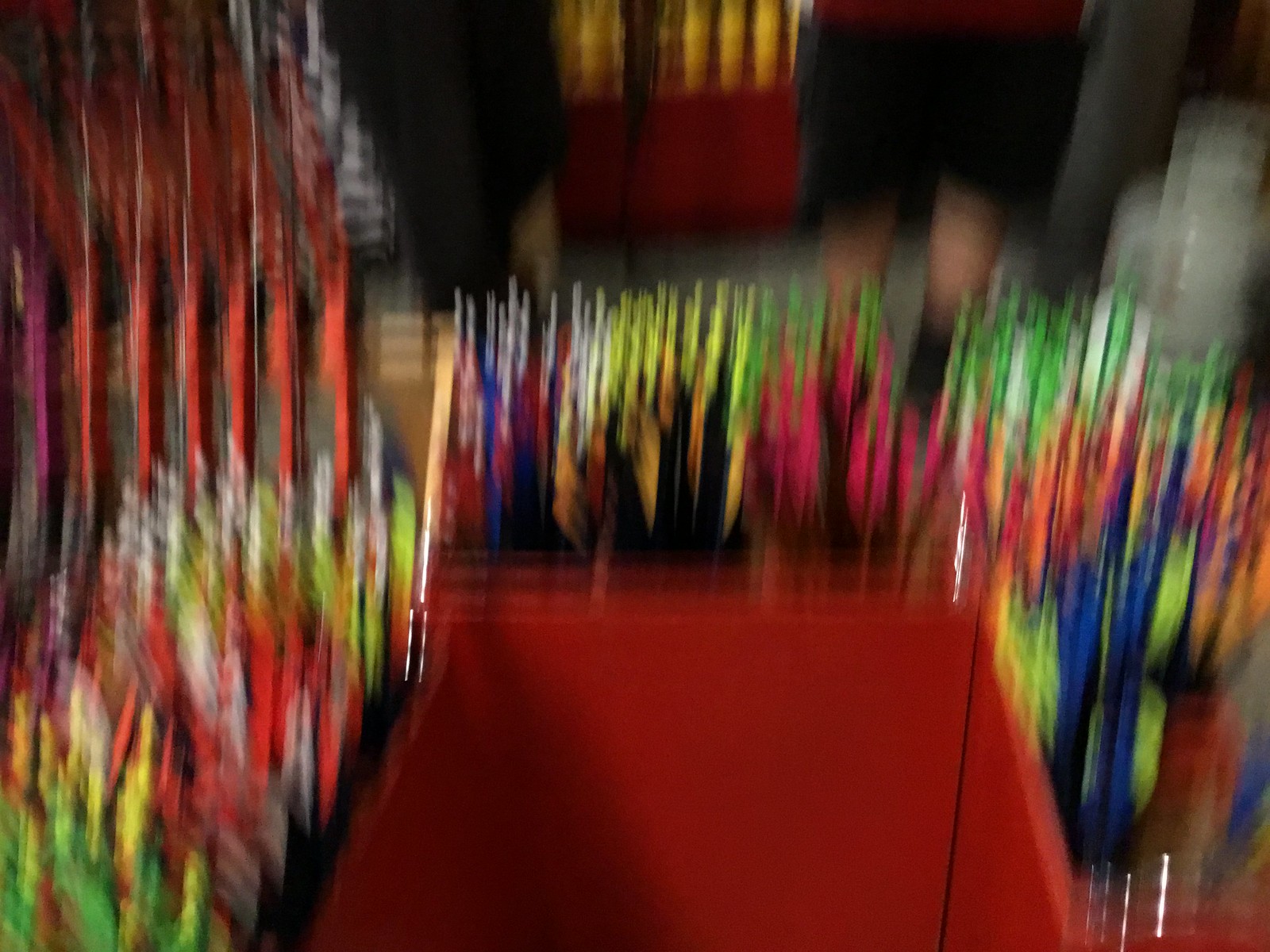This image, whether a color photograph with a deliberate blur effect or a painting with expressive brush strokes, features an abstract scene rich in color and form. At the very bottom, a maroon square anchors the composition. To the left of this square, a vibrant cluster of colors emerges, blending lime green, yellow, pink, bright red, white, and gray in a dynamic, swirling pattern. This amalgamation of hues suggests either an artistic photo effect or the textured strokes of a painting. Above this colorful mass rise several tall, pole-like structures in a similar reddish maroon shade, adding vertical movement to the scene. Behind the maroon square, more colorful figures extend into the background and repeat on the right side, creating a harmonious balance of chaotic color. The overall effect is a captivating blend of form and color, inviting viewers to interpret its abstract nature.